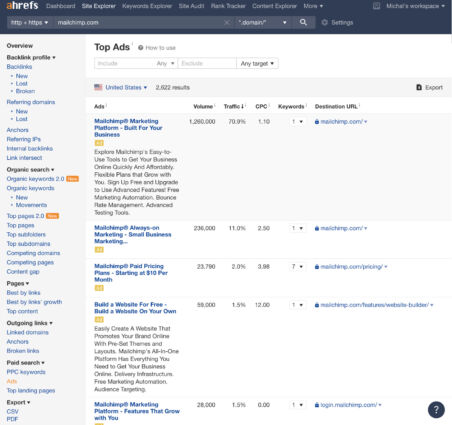The image depicts a webpage interface, specifically from the Ahrefs site. The top of the page features a dark blue bezel. Positioned on the left side of the bezel is an orange "A," followed by the text "HREFS" in white. 

The navigation bar includes several tabs: "Dashboard", "Site Explorer" (which is selected and highlighted in bright white), "Keyword Explorer," "Site Audit," and another tab that's partly blurred but appears to be "Plank something." Other tabs include "Contact Explorer" and "More," the latter featuring a down arrow for a dropdown menu. Additionally, there is a section labeled "Michael's workplace," indicated with a calculator symbol, though the name "Michael" is either mispronounced or misspelled as "M-A-C-H-E-L" or "A-L."

Below the navigation bar, there is a gray sidebar on the left-hand side of the page with a detailed list: 

- "Overview" in bold black
- "Backlink Profile" also in bold black, followed by:
  - "Backlinks"
  - "New"
  - "Lost"
  - "Broken"
  - "Referring Domains," followed by:
    - "New"
    - "Lost"
  - "Anchors"
  - "Referring IPs"
  - Additional blurred items, one of which starts with "Link"

The list continues within the organic search section, featuring:
- "Organic Search" in black, followed by items in blue hypertext:
  - "Organic Keywords 2.0"
  - "Organic Keywords," then
  - "New," followed by another "New" item that is partly blurred
  - "Top Pages 2.0"
  - "Top Pages"
  - "Top Subfolders"
  - "Top Subdomains"
  - "Comparing Domains"
  - "Competing Pages"
  - "Content PHP"

Further down, under "Pages," black text is labeled with a dropdown triangle.
- Below are blue hypertext links:
  - "Best By Links"
  - "Best By Links Growth"
  - "Top Content" or "Top Comment"

Next, an outgoing links section, highlighted in black, is followed by:
- Blue hypertext links:
  - "Link Domains"
  - "Anchors"
  - "Broken Links"

Under "Paid Search," also labeled with a dropdown arrow, blue hypertext includes:
- "PPC Keywords"
- In orange text: "APTS"
- Followed by another blue hypertext: "Top Landing Pages"

The next section, highlighted in black with a down arrow, reads "CSV and PDF."
- Additional blurred webpage elements, most recognizable as "MailChimp," are shown against a white background.